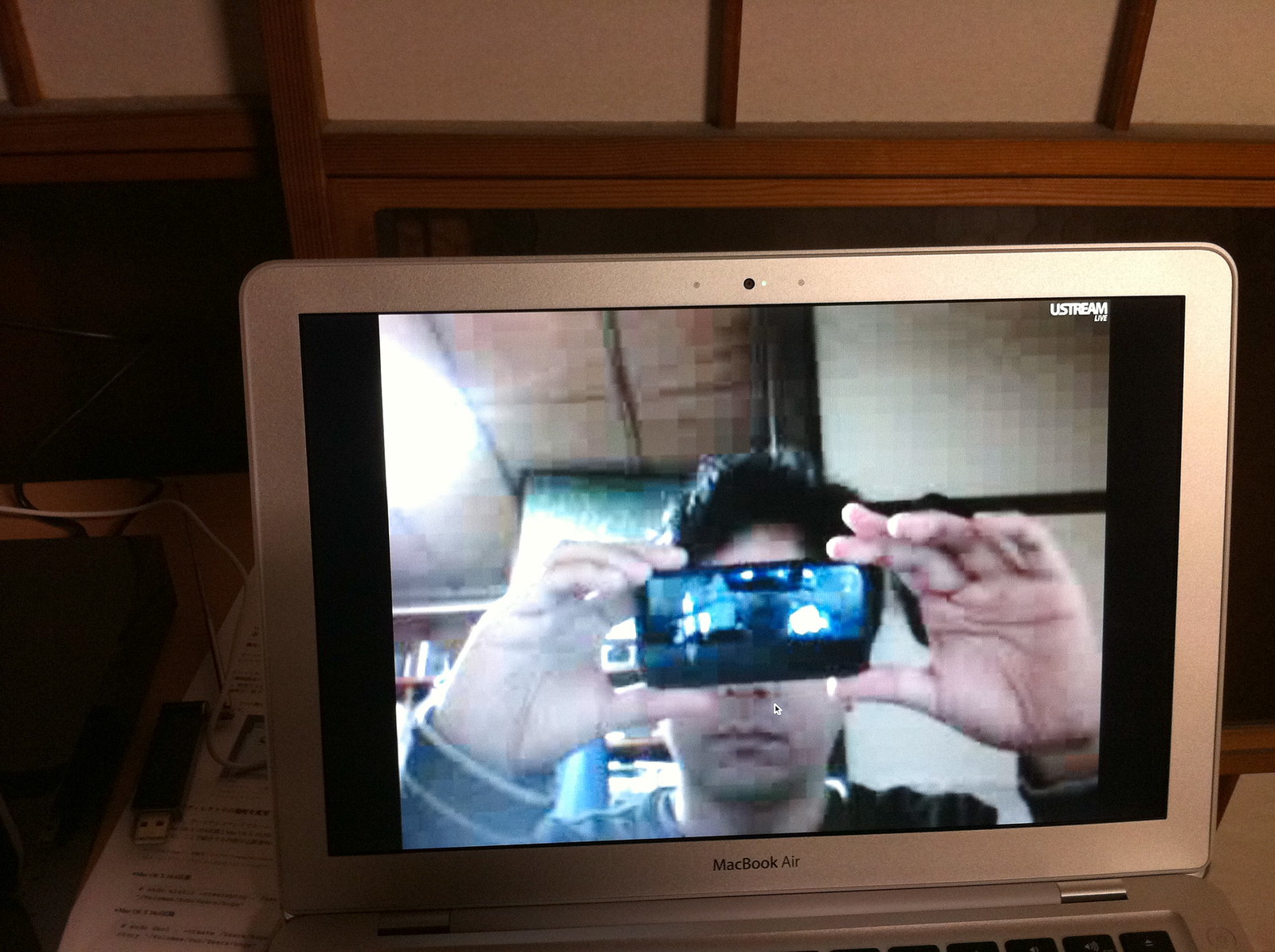The photograph captures a minimalist scene featuring a silver MacBook Air, which is largely cut off, displaying a live stream via Ustream. The visible part of the laptop shows a tiny sliver of its black keyboard and the iconic "MacBook Air" text at the bottom of the built-in monitor. Central to the image is the computer screen, which portrays an Indian man with dark hair, clad in a green sweater, holding up a smartphone toward the camera. The phone's screen indicates that the laptop is recording him. The man’s hands are prominently visible as he presents the device. Adding to the scene, a USB drive and some scattered white papers are placed on the table beside the laptop, anchoring the setup in a lived-in workspace.